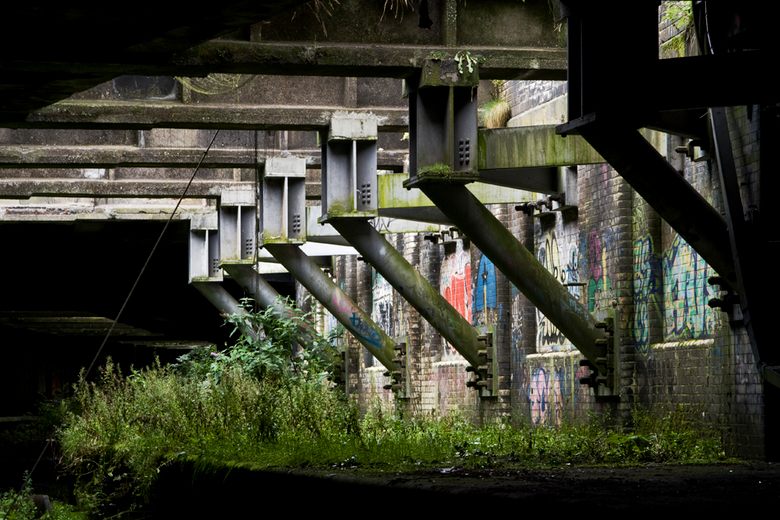This photograph, taken at nighttime, captures the underside of a bridge or overpass, revealing a complex structure with steel support beams bolted into a brick foundation. The brick walls, now covered in random graffiti, exhibit signs of decay, including mold, moss, and rust on the metal beams. Despite the wall being well-lit, the entire scene is tinged with darkness, emphasizing the neglected nature of the area. Overgrown vegetation, consisting of reeds, bushes, and a small tree, occupies the ground beneath the structure, adding to the abandoned feel. The image primarily focuses on the right side of the structure, with no visible background details due to the pervasive darkness, hinting at the bridge's location possibly near a canal in an inner city.